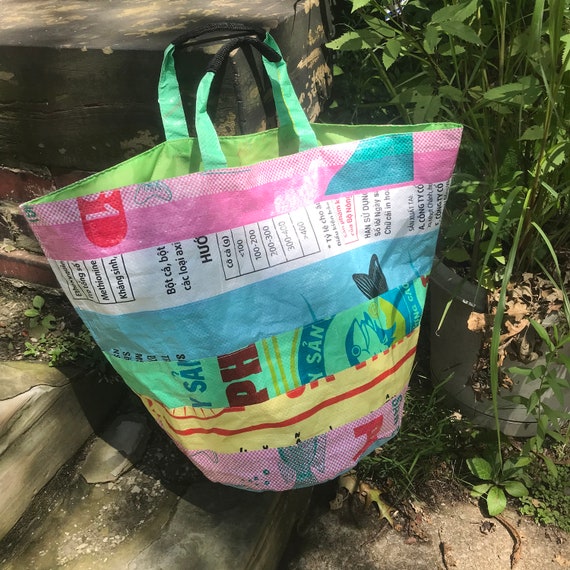This outdoor photograph features a prominent, multi-colored tote bag made from recycled materials, hanging off the top step of a concrete stoop. The bag displays an eclectic patchwork design, consisting of vibrant layers: a top pink section with red and teal shapes, followed by a white layer with black, sideways text, possibly in an Asian language. Further down, there are blue, green with brown, yellow, and blue text, yellow with red, and another pink layer. The interior of the bag is lime green, paired with mint green handles that have black grips at the top. Surrounding the stoop, a variety of green plants with leafy stems add a natural backdrop, spilling over to the right and partially obscuring the scene. The overall image captures a blend of urban and natural elements, with the sturdy, weathered steps and flourishing greenery framing the colorful focal point of the reusable tote.